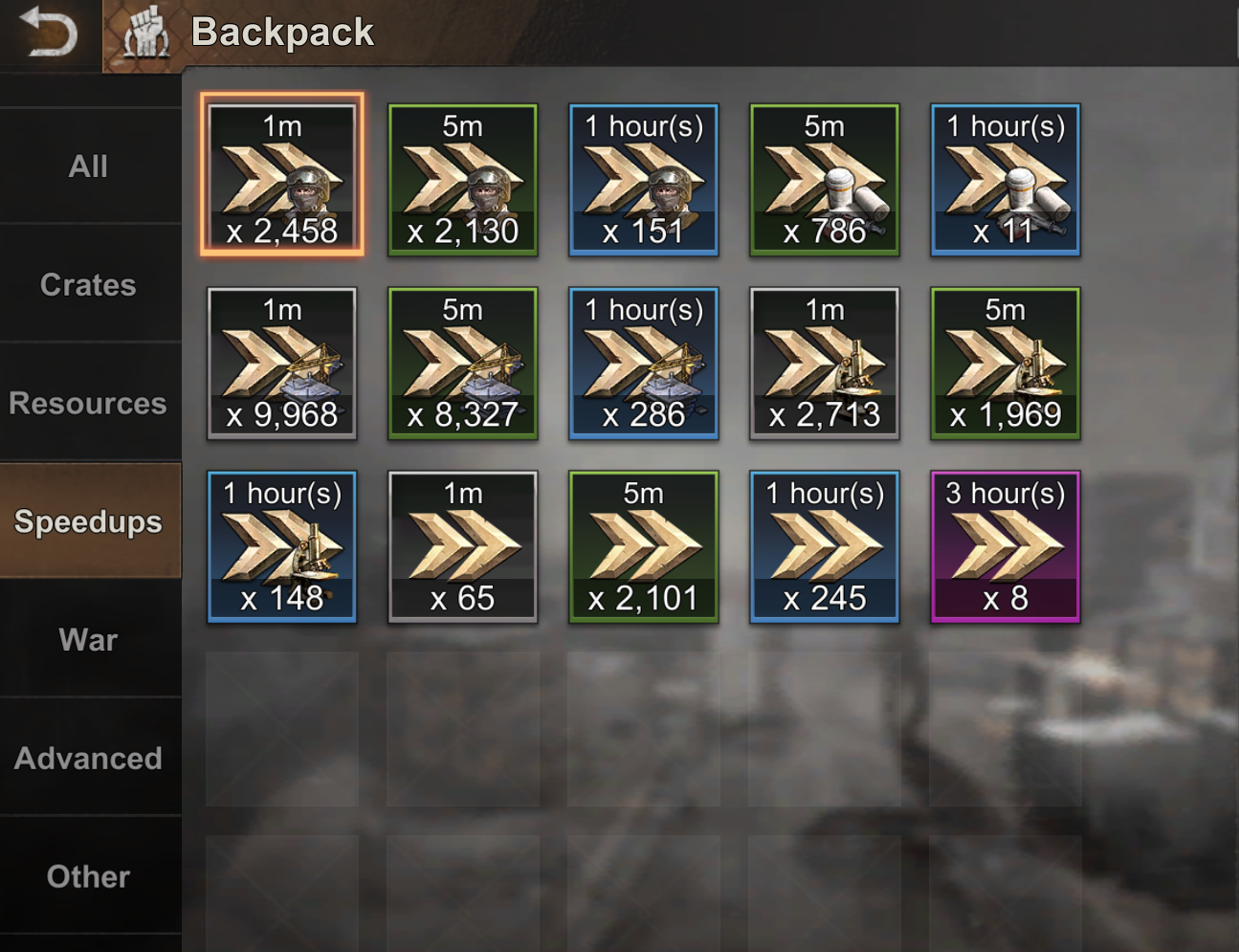This image is a detailed screenshot from a video game interface, specifically an inventory or resource management menu labeled "Backpack." The interface is indicative of a strategy or role-playing game where resource management is crucial. In the upper left-hand corner, there is a curved arrow icon next to a raised fist icon, followed by the word "Backpack" in white letters. 

On the left side of the interface, there's a vertical navigation menu with tabs labeled "All," "Crate," "Resources," "Speedups," "War," "Advanced," and "Other." The "Resources" tab is currently highlighted, suggesting the items displayed belong to this category. 

The main part of the interface features a grid layout comprising three rows with five squares in each row. Each square contains an icon, often depicting an arrow and a man in a helmet, along with quantities and a time designation such as "1M" or "5M." For example, one item is shown with the text "1M" over an icon of an arrow and a man in a helmet, with "X2,458" listed below, indicating the player possesses 2,458 units of this item. Another item shows "5M" with the same icon and "X2,130" below it.

This layout and detailed labeling suggest a sophisticated system for managing various in-game resources efficiently.